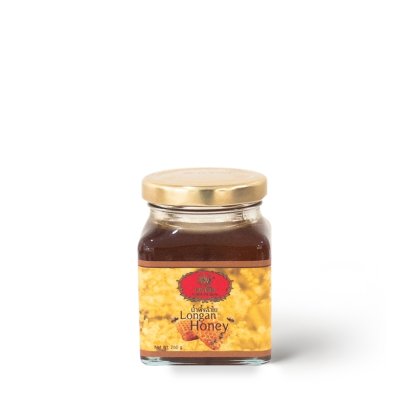The photograph depicts a professionally taken studio image of a small jar of Longan Honey set against a pristine white background devoid of shadows. The jar, made of glass, is square-shaped and transitions into a round shape at the top where it has a gold-colored, screw-on lid. Inside, the honey is a rich, deep amber color. The jar's label is primarily yellow with a thin gold band at the top and bottom. It prominently features the words "Longan Honey" and includes additional text that appears to be in Arabic or Indian script. Above the text, there is a red and brown logo that is somewhat blurred or difficult to read. The label also contains net weight information that is not clearly legible.